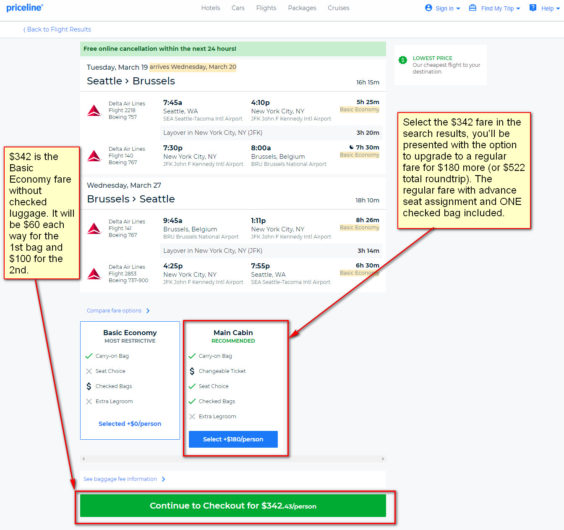This is a detailed screenshot from the Priceline website, showcasing a flight search result for a trip from Seattle to Brussels. The top navigation bar includes options for hotels, cars, flights, packages, cruises, sign in, find my trip, and help. Below this, there is a "Back to flight results" link and a banner highlighting "Free online cancellation within the next 24 hours" in a green field.

The search result details a round-trip flight departing on Tuesday, March 19th, arriving on Wednesday, March 20th. Both flights are operated by Delta Airlines. 

- **Outbound Flight:**
  - Leg 1: Departs Seattle at 7:45 AM, arriving in New York at 4:10 PM (Duration: 5 hours 25 minutes).
  - Layover: 3 hours and 20 minutes in New York.
  - Leg 2: Departs New York at 7:30 PM, arriving in Brussels at 8:00 AM the next day (Duration: 7 hours 30 minutes).

- **Return Flight:**
  - Leg 1: Departs Brussels at 9:45 AM, arriving in New York at 1:11 PM (Duration: 8 hours 26 minutes).
  - Layover: 3 hours and 14 minutes in New York.
  - Leg 2: Departs New York at 4:25 PM, arriving in Seattle at 7:55 PM (Duration: 6 hours 30 minutes).

The search results offer both Basic Economy and Main Cabin options, with the Main Cabin being recommended at $180 per person. A red rectangle and an arrow highlight this recommended option within the screenshot, pointing to a text field that instructs to select the $342 fare in the search results. This will present the option to upgrade to a regular fare for an additional $180, totaling $522 round trip. The regular fare includes advanced seat assignment and one checked bag.

At the bottom of the screenshot, a green button labeled "Continue to checkout for $342.43 per person" is shown. Adjacent to this button, a red arrow calls out an explanation: "$342 is the basic economy fare without checked luggage, with an additional $60 each way for the first bag and $100 for the second bag."

This screenshot has multiple call-outs to guide the user through the selection and payment process, emphasizing the costs and benefits of upgrading to a regular fare.